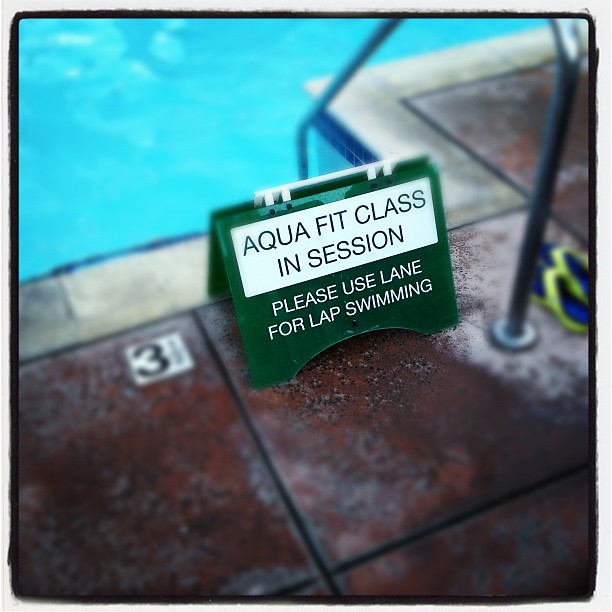The photograph captures a close-up view of the entrance to a swimming pool, featuring a triangular, foldable green placard prominently placed near the pool's edge. The placard, which has a white section at the top, announces in bold text "AquaFit class in session" and instructs, "please use lane for lap swimming" below. This sign is situated near a set of descending stairs, which are partially visible in the image along with a shining chrome handrail to the right. The floor around the pool consists of large, heavily pitted, reddish-brown stone tiles with defined black grout lines in between. A number "3" on a white square is embedded in one of the tiles to the left of the placard, while the light blue water of the swimming pool provides a serene background, completing the evocative scene.